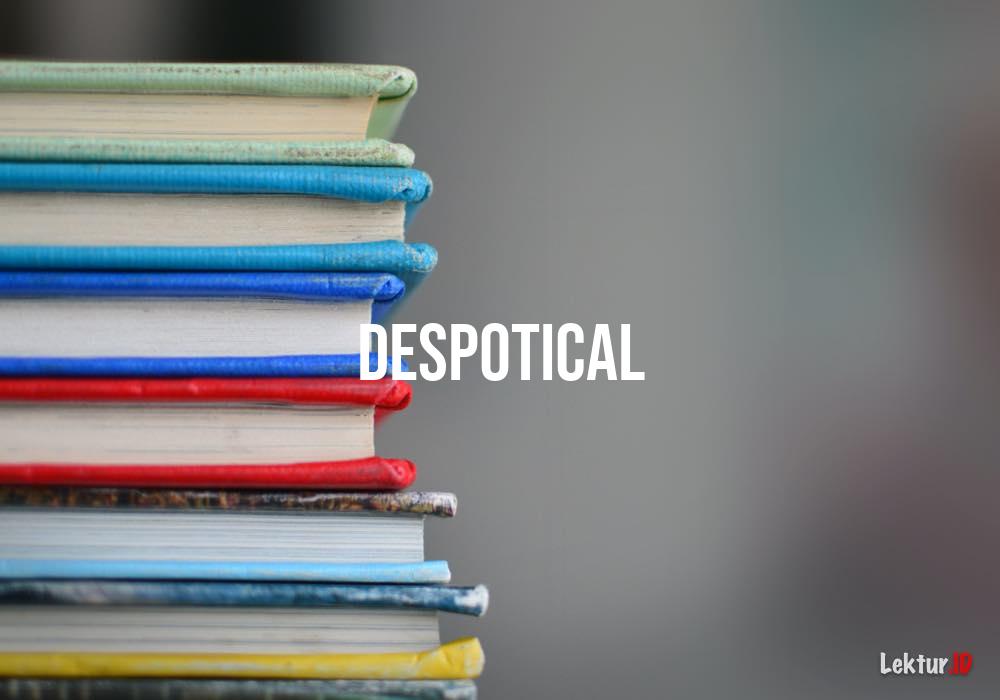The image showcases a stack of six thin books, all oriented towards the left side of the frame. The books, each featuring white pages and different colored bindings, are neatly piled on top of one another. The colors of the book covers from top to bottom are mint green, light blue, dark blue, red, brown with possible baby blue elements, and yellow. The left-aligned stack leaves the right side and center of the photo uncluttered, highlighting a central piece of text that reads "DESPOTICAL" (spelled D-E-S-P-O-T-I-C-A-L). In the bottom right corner, there is a logo that reads "Lector.id" with "Lector" rendered in white and "id" in red. The background of the image is heavily blurred, reducing it to indistinct gray and colored blobs, which lends a focused prominence to the books and text, suggesting the scene might be part of a presentation slide.